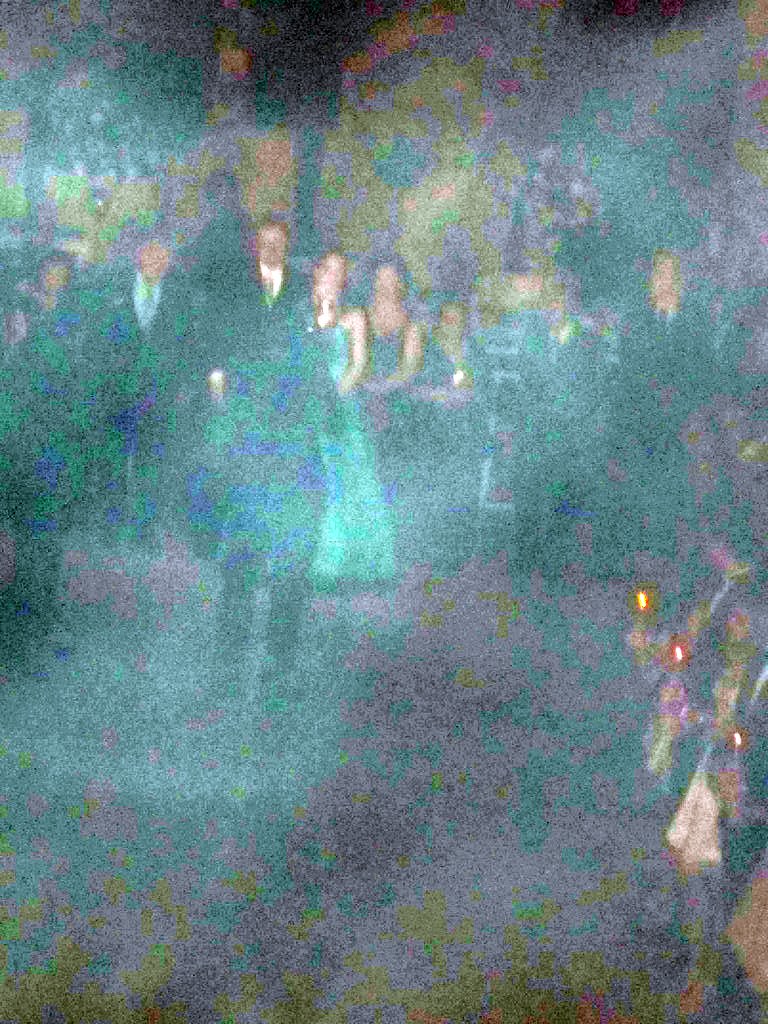A blurred and low-quality image captures a formal event in a darkened room. Despite the lack of clarity, the scene depicts numerous attendees in elegant attire, with men in suits and women in ball gowns. The configuration suggests it could be a wedding, prom, or similar formal gathering. Along the back wall, several individuals can be seen, while others are positioned at right angles along the side of the frame. The image lacks further detail but conveys the ambiance of a grand occasion attended by formally dressed guests.